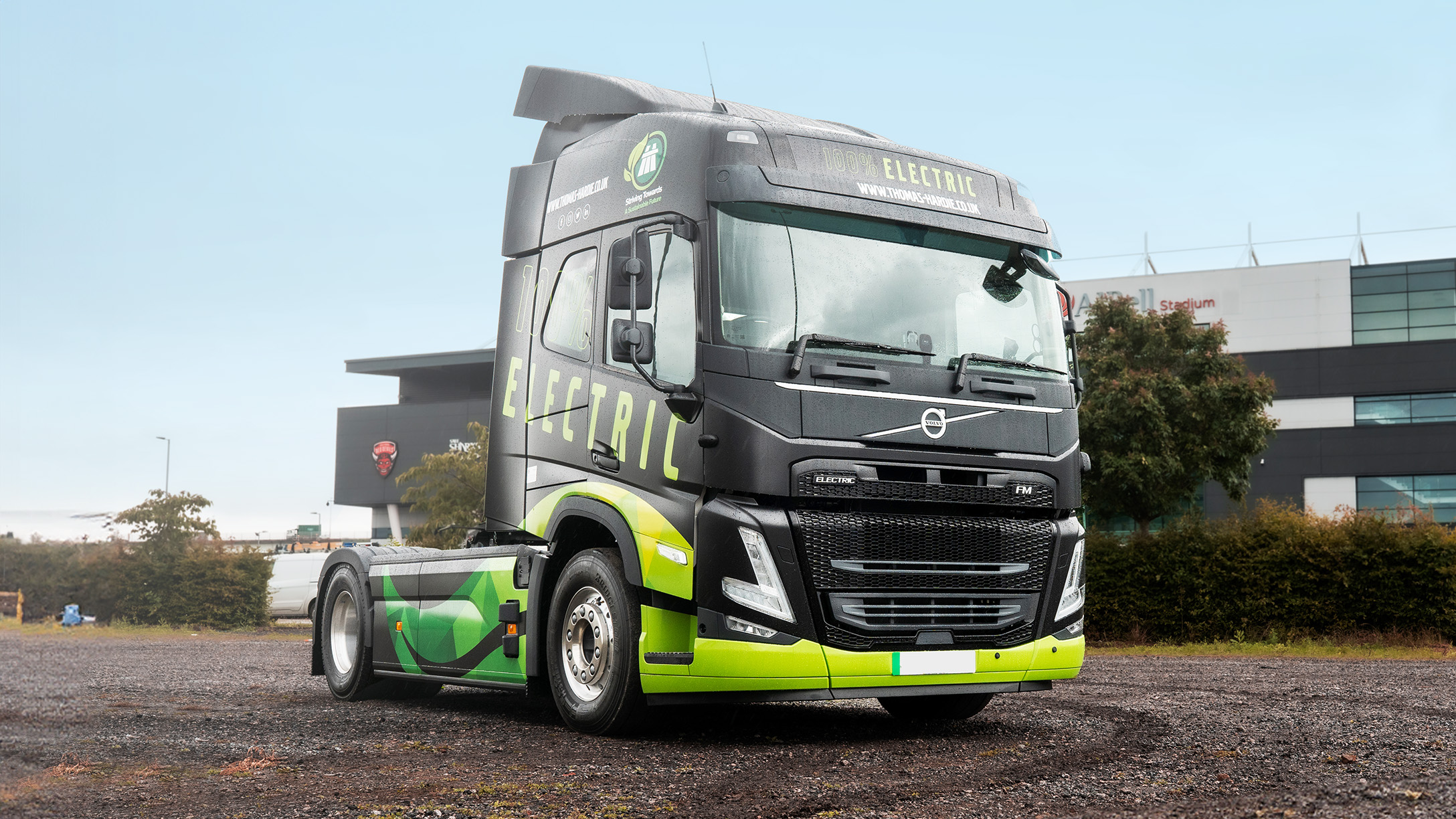The image features a close-up of a brand new, electric-powered Volvo semi-truck, prominently positioned as if advertised for sale. The truck, centered in the photo, boasts a sleek black cab accented with vibrant green graphics that transition from medium green on the sides to a striking lime green at the front. Notable text reading "electric" can be found on the right-hand door and above the windshield, hinting at its eco-friendly design. The truck's cab is characterized by a flat front grille and windshield, along with an air dam on the roof, suggesting aerodynamic efficiency for hauling trailers. It is parked in a gravel yard with brown-gray ground, against a backdrop of a modern building and some hedges. The sky is a clear, light blue, complementing the clean and polished appearance of the vehicle, which even shows subtle water droplets on its roof, indicating its pristine, just-detailed condition.